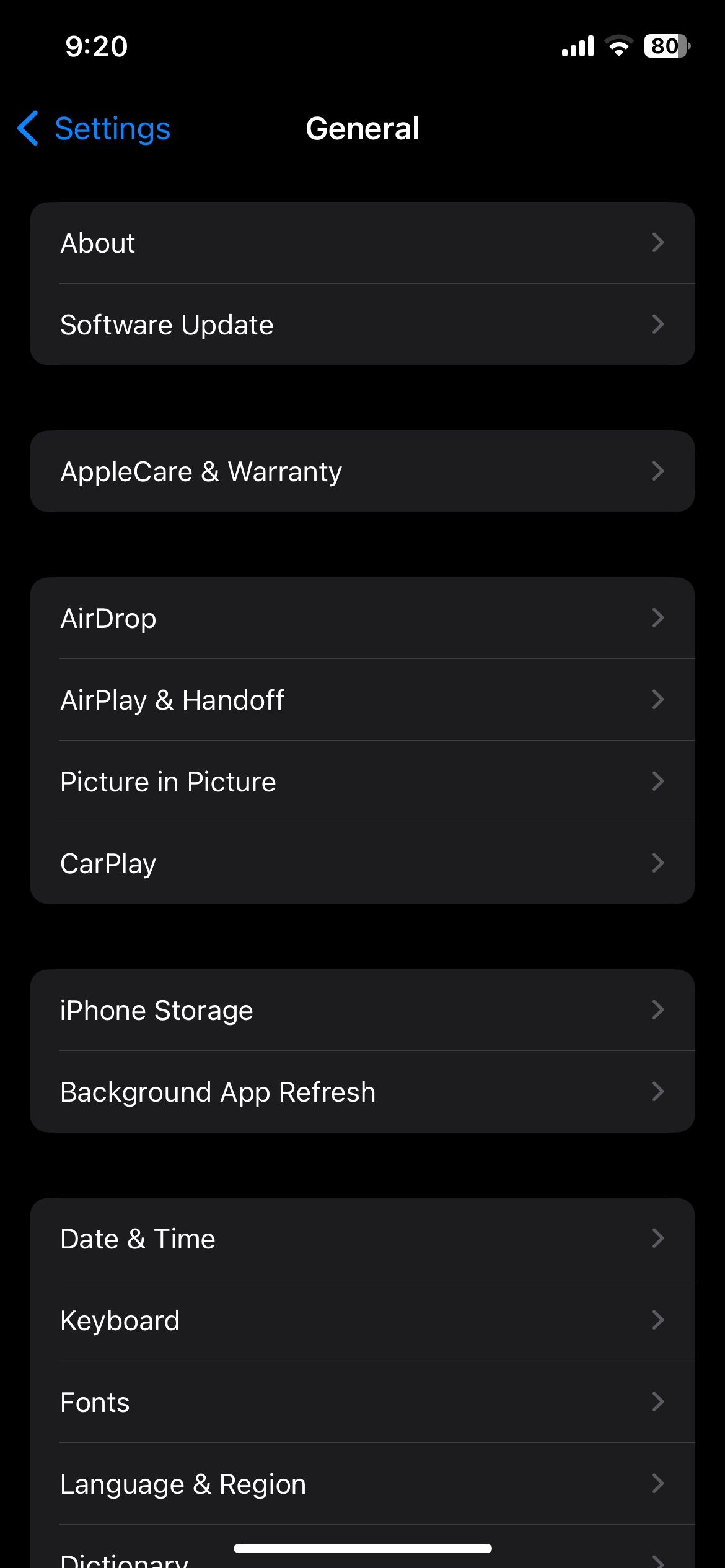The image displays a smartphone screen against a black background. In the top left corner, the UI shows the current time as 9:20, with indicators for four cellular bars, a half-filled Wi-Fi signal, and an 80% battery life. Below this, a blue arrow points to the left beside the word "Settings," indicating navigation options.

Centered on the screen is a section titled "General," with text in white. Directly beneath this heading is a gray box containing the options "About" and "Software Update." Following this, another gray box lists "AppleCare and Warranty," highlighted by a gray arrow pointing to the right.

Next, a larger gray box encompasses several settings: "AirDrop," "AirPlay and Handoff," "Picture in Picture," and "CarPlay," each followed by a right-pointing gray arrow. Further down, a new gray box begins with "iPhone Storage" at the top, paired with a right-side arrow, and includes the option "Background App Refresh" below it.